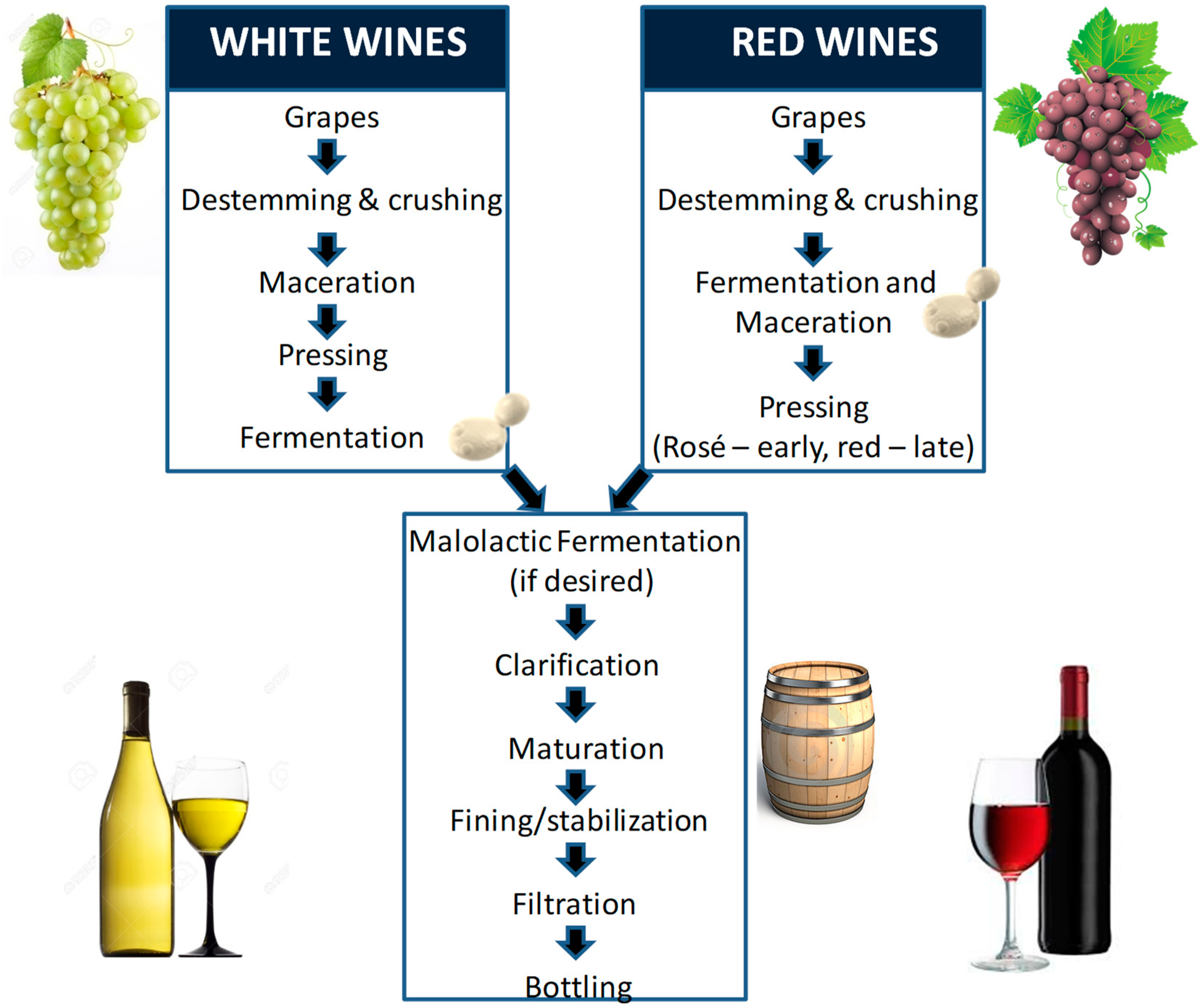This image illustrates the comprehensive process of winemaking, featuring both white and red wines. On the left, a chart detailing the production of white wine begins with green grapes, followed by de-stemming and crushing, progressing through maceration, pressing, and then fermentation. Adjacent to this chart is an image of fresh green grapes. On the right, a similar chart outlines the red wine production process, starting with red or purple grapes, moving through de-stemming and crushing, followed by fermentation and maceration, then pressing - with rosé wines pressed early and red wines pressed later. This chart is accompanied by an image of red grapes with green leaves.

Both charts converge into a third one at the bottom, depicting the final stages common to both wine types: optional malolactic fermentation, clarification, maturation, fining, stabilization, filtration, and finally, bottling. This chart is complemented by several photographic elements: on the left, a bottle of white wine and a half-filled glass of white wine, and on the right, a barrel and a bottle of red wine with a half-filled glass of red wine. The entire visual is a blend of computer-generated graphics and photographic icons, giving a detailed, step-by-step depiction of the winemaking process from grape selection to bottling.